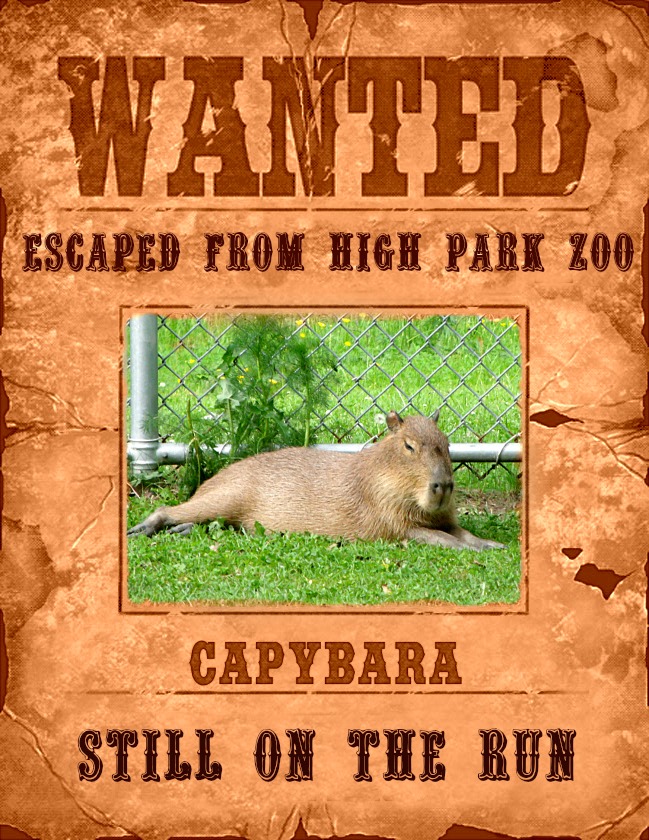This image features a humorous wanted poster styled after the Old American West, with bold brown letters proclaiming "WANTED" at the top. Below that, in black text, it states "ESCAPED FROM HIGH PARK ZOO." The centerpiece of the poster is a photograph of a capybara, depicted lounging on green grass with a backdrop consisting of a cyclone fence and a small, newly sprouted pine tree. Beneath the photograph, the word "CAPYBARA" is spelled out in brown letters, followed by "STILL ON THE RUN" in black text at the very bottom. The background of the poster has been digitally rendered to resemble old, cracked, and discolored tan paper, laid out as if pasted onto wood, enhancing its vintage aesthetic. The capybara, which looks somewhat like a dog-sized rodent with a distinctive, pronounced nose, adds a whimsical touch to the overall design.